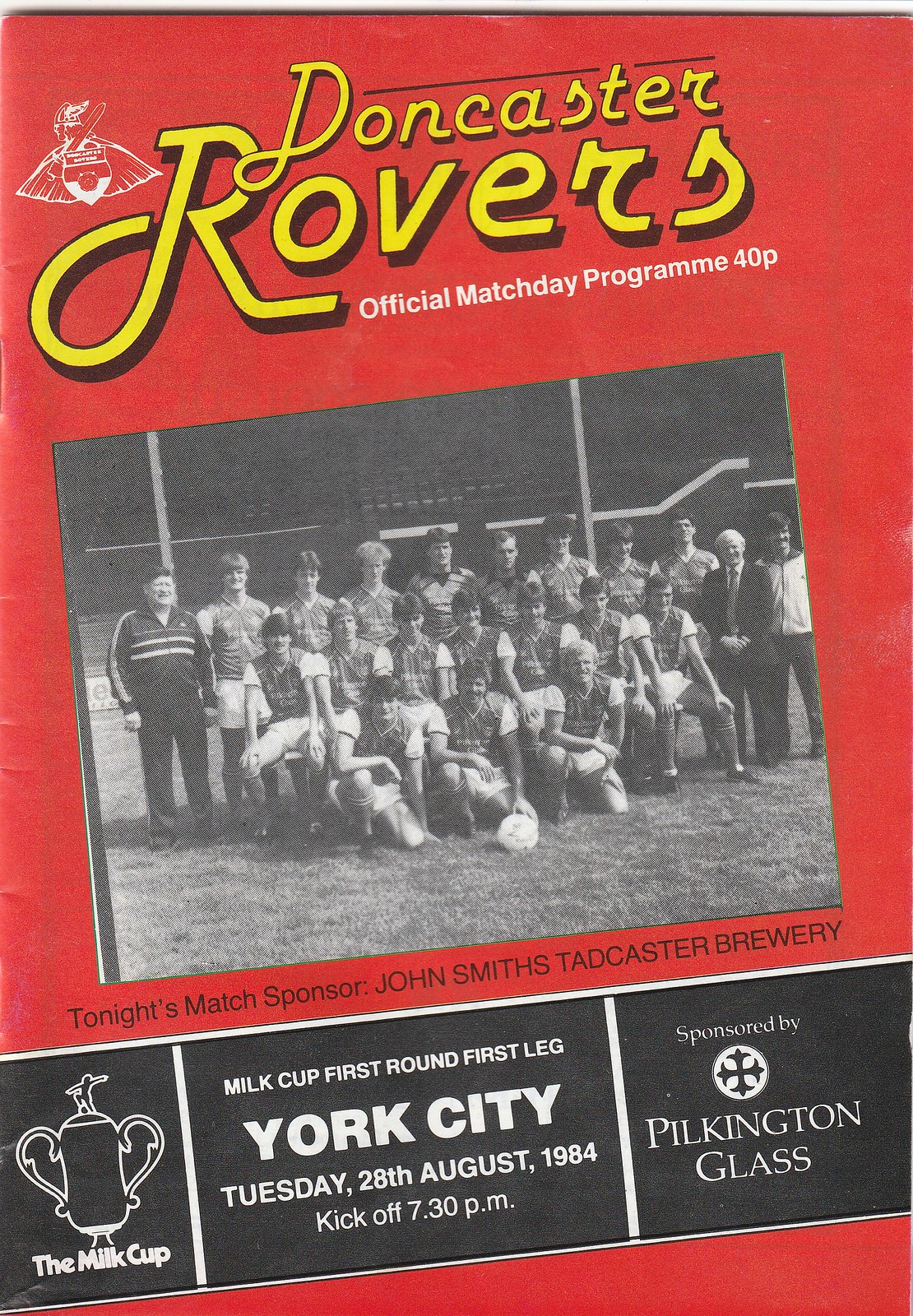The image displays the cover of an official matchday program for the Doncaster Rovers. The background is predominantly red with "Doncaster Rovers" spelled out in yellow letters at the top. Below this, in white text, it reads "Official Matchday Program 40p." A white team logo is placed in the top left corner. Centrally, there is a slightly tilted black-and-white team photo showing about 15 young players and a few coaches; the frontline players are leaning on their knees, with one player in the middle holding a soccer ball with his left hand. Beneath the photo, the text indicates "The Milk Cup" along with its trophy image, followed by details of the match: "Milk Cup First Round, First Leg York City, Tuesday 28th August 1984, Kickoff 7.30 p.m." Also noted is the sponsorship by "John Smith's Tadcaster Brewery" and "Pilkington Glass," in white text on a black background at the bottom. The image is both promotional and informative, capturing the essence of a historical sports event.